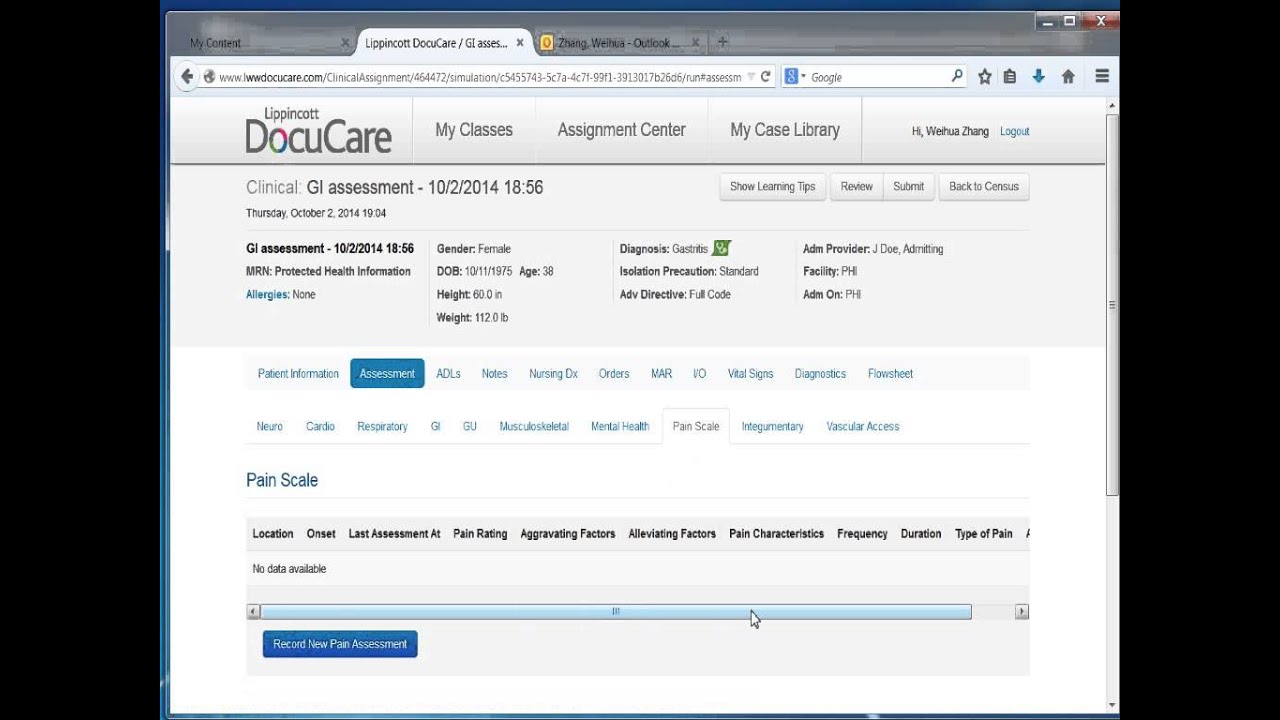This detailed screenshot captures an open browser window with three tabs, where the center tab is currently selected. The URL is prominently displayed in gray and black text underneath the tab. Dominating the bottom-left portion of the screen is the company logo, featuring the name 'Lippincott' with 'DocuCare' written below.

Navigating the top menu, there are several clickable links: 'My Classes,' 'Assignment Center,' 'My Case Library,' and a greeting to the user on the far right, along with a blue 'Logout' button. The background color is primarily light gray, with a central white section featuring extensive blue text detailing patient information and assessments.

Highlighted in this section is the word 'Assessment,’ presented with white writing on a blue background. Next to it, in blue text, are entries such as 'ADLs,' 'Notes,' 'Nursing DX,' and 'Orders,' among others, indicating various patient information categories.

Further down, a dark blue title reads 'Pain Scale,' followed by different categories describing the patient's pain, including location, onset, last assessment, pain rating, aggravating and alleviating factors, pain characteristics, frequency, duration, and type of pain. At the very bottom, there is a blue rectangular button labeled 'Record New Pain Assessment' in white text.